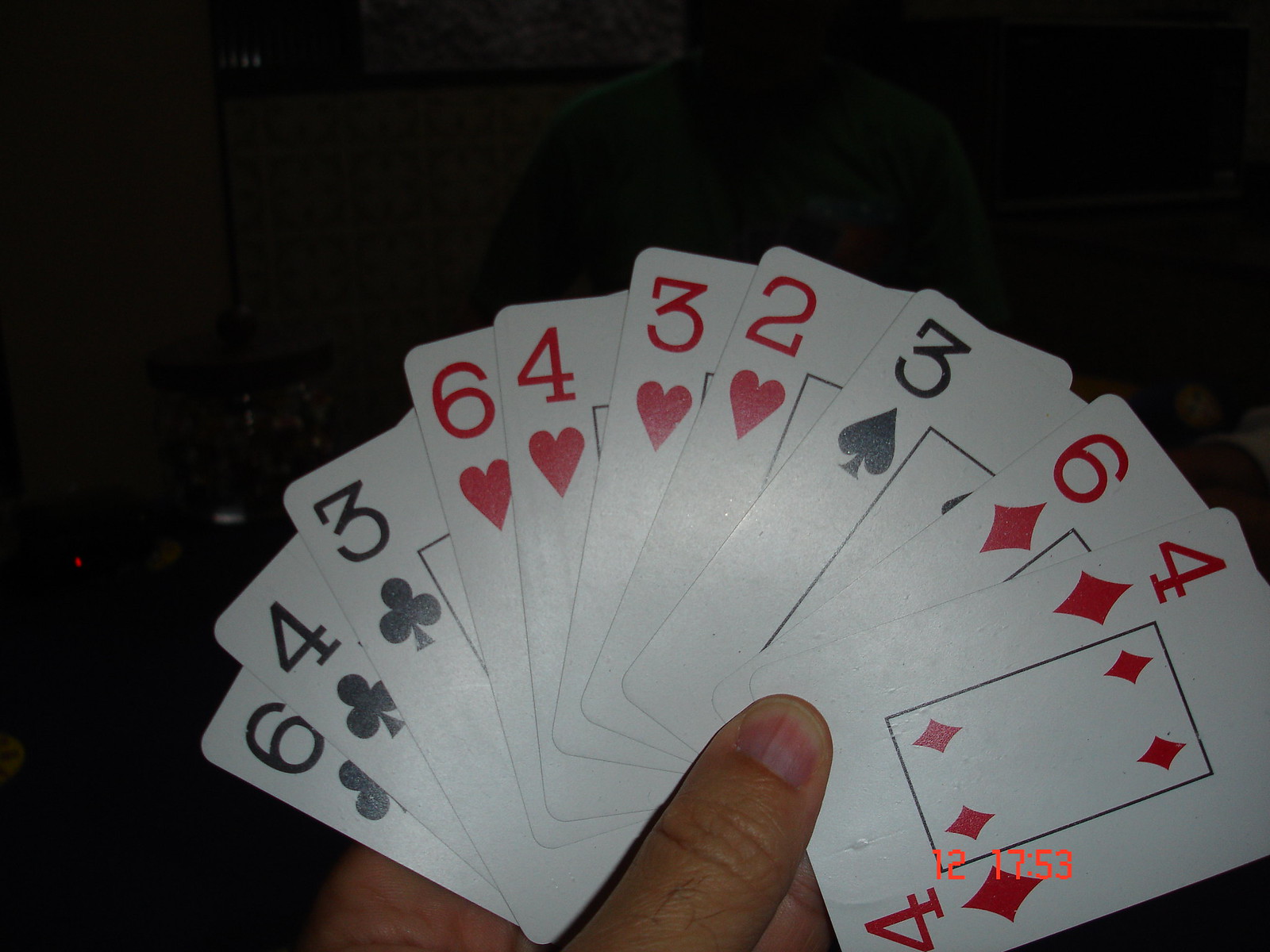A detailed photograph captures a hand delicately holding an array of playing cards against an almost pitch-black background speckled with faint red and white lights. In the bottom right corner, a red digital timestamp reads "1217:53," reminiscent of an image taken on a digital camera. The person holding the cards has dark brown skin, and their thumb is visible, showcasing a very small fingernail. The cards are faned out in an arc, from the bottom-most card on the left to the top-most on the right. The displayed cards include a six of clubs, four of clubs, three of clubs, six of hearts, four of hearts, three of hearts, two of hearts, three of spades, six of diamonds, and four of diamonds. Each card is white, adorned with large black and red numbers and symbols. Centrally, a black, skinny, outlined rectangle on each card encloses the respective suits' symbols, enhancing the visual appeal against the stark darkness.